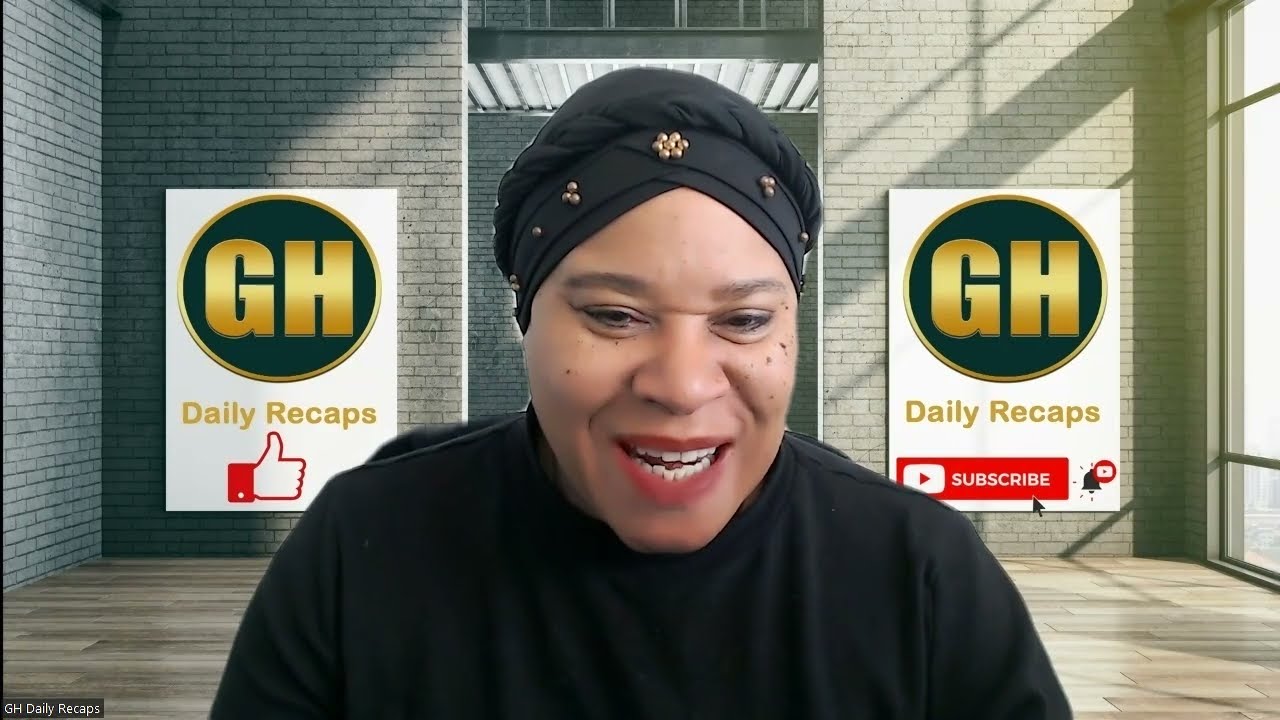In front of an industrial-themed space, featuring light brown wooden floors and a grayish brick wall, stands a woman dressed entirely in black. She wears a black sweater and a black hat, which resembles a turban adorned with gold beads on the side. Her red lipstick stands out as she smiles and appears to be talking. Behind her, the brick wall displays two white rectangular posters. Each poster has a black circle with a gold outline and the capital letters "GH" in gold. Below these, the phrases "daily recaps" and a thumbs-up symbol are present. To her left is a floor-to-ceiling window through which light is streaming, and on the right side, there is another poster featuring a "subscribe" rectangle.